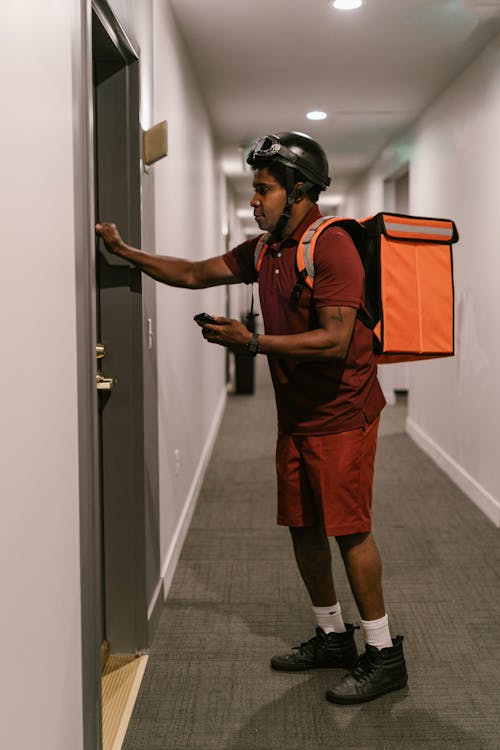In this image, a brown-skinned food delivery man is depicted knocking on a door in what appears to be an apartment building hallway. He is dressed in a maroon polo shirt and red knee-length shorts, complemented by white socks and worn black high-top sneakers. A large, square, and reflective orange food delivery backpack is strapped to his back, suggesting he is carrying food, possibly a pizza. He wears a black helmet with attached black goggles for protection, likely indicative of him riding a bicycle, moped, or motorcycle.

In his left hand, he holds a cell phone and wears a watch, while his right hand is raised in the act of knocking on a dark gray door. The hallway features light gray walls, a gray carpet, and a white ceiling equipped with circular lights evenly spaced along its length. The overall setting hints at a residential complex, with multiple doors lining the corridor.